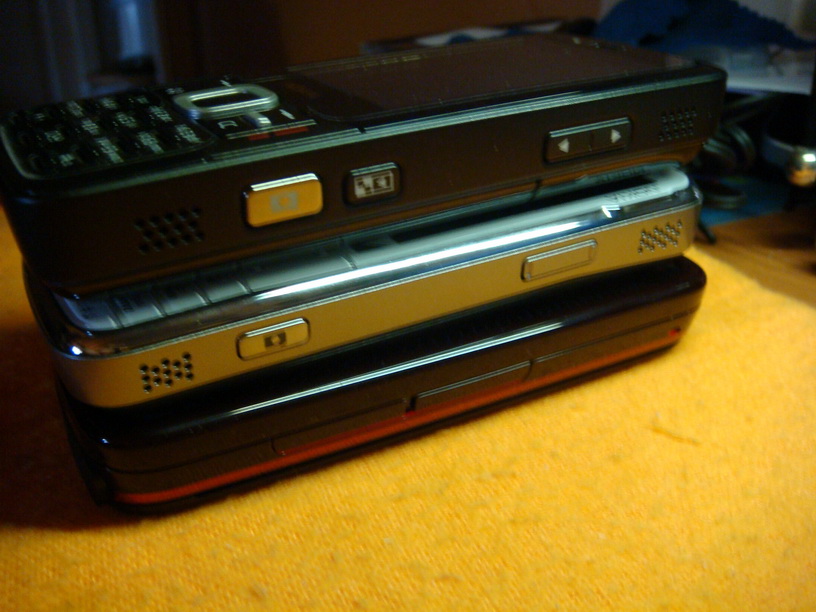The image depicts a close-up, slightly grainy and out-of-focus photograph of three old-fashioned, brick-style cell phones stacked on a yellow tablecloth or rug. The stack is composed of three distinct phones: at the bottom is a black phone with a red stripe and buttons visible on the side and front; in the middle is a silver phone with a grey plastic face and keypad; and on the top is a chunky black cordless handphone with a standard keypad featuring ABC123 input. The setting includes an orange tabletop or counter, with a backdrop of more indistinct items, a doorway, and possibly a car windshield, adding depth to the scene. The photograph, while low resolution, provides a nostalgic view of these large and bulky devices, once commonly referred to as "bricks."